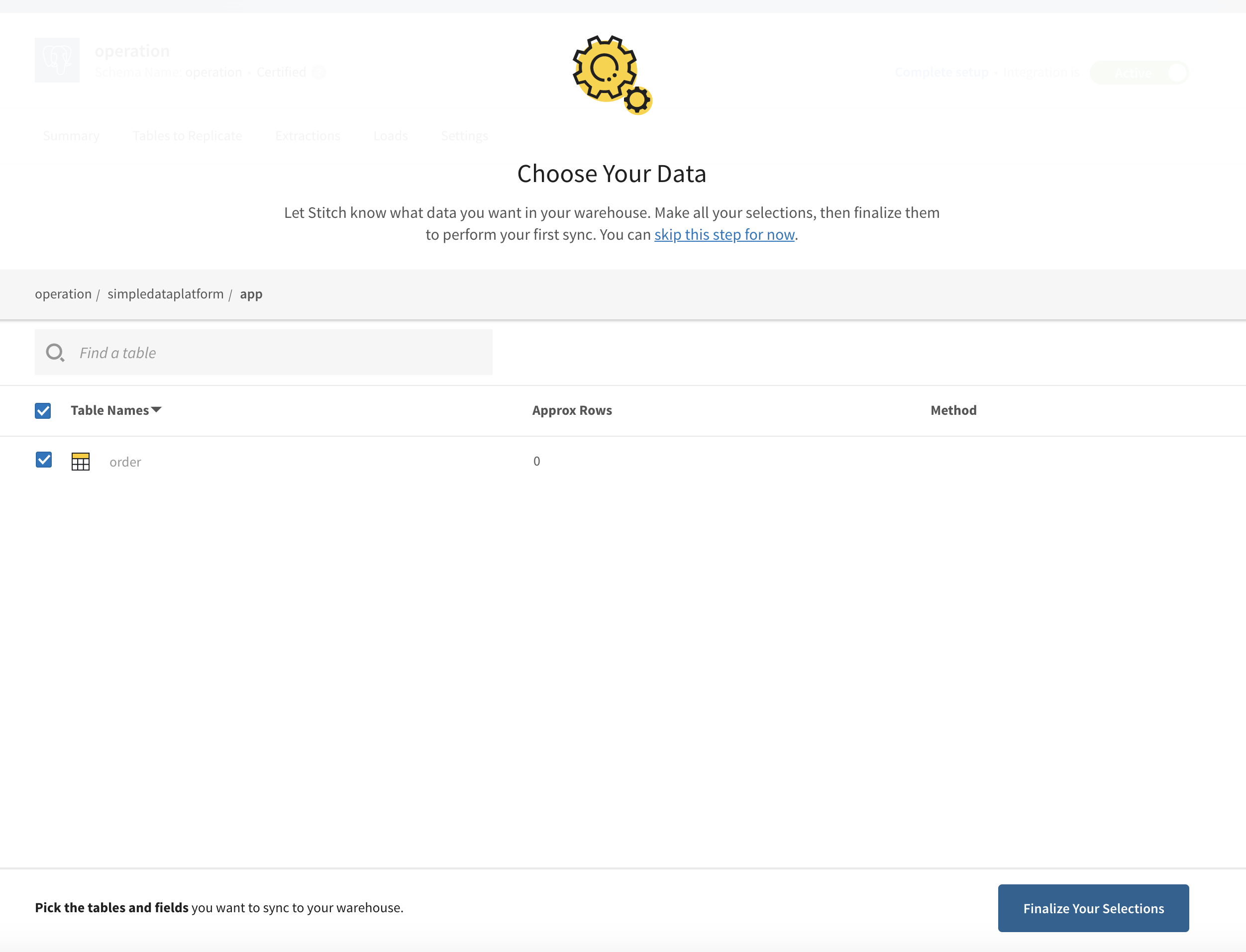The image appears to be a screenshot from an unfamiliar application with a predominantly white background and black text interspersed with small icons. 

### Top Section:
- **Cogwheel Icon:** Located at the top of the image are two cogwheels, one large and one small, highlighted in yellow.
- **Header Text:** Below the cogwheel icon, the text reads "Choose Your Data" in bold, followed by "Let Stitch know what data you want in your warehouse. Make all your selections then finalize them to perform your first sync. You can skip this step for now."
  - **Link:** The phrase "skip this step for now" is highlighted in blue and underlined, indicating it is a clickable link.

### Middle Section:
- **Gray Bar:** Beneath the instructional text, there is a horizontal gray bar with the following path: "operations / simpledata platform / app operations simple data platform / app."
- **Search Bar:** Directly below the gray bar is a search bar with a placeholder text reading "Find a table," suggesting the user can type in any query.
  
### Main Section:
- **Options:** Below the search bar, there are two options displayed as checkboxes, both checked and turned blue:
  - **Table Names:** Accompanied by a dropdown menu.
  - **Calendar:** Denoted by a calendar icon, labeled "Order."
  - **Columns:** The table columns include "Table Names," "Aprox Rows," and "Method."
    - Next to "Calendar" under "Aprox Rows," it reads "0" and the "Method" column is blank.

### Bottom Section:
- **Instructional Text:** "Pick the tables and fields you want to sync to your warehouse."
- **Finalize Button:** In the bottom right corner, there is a blue button labeled "Finalize your selections."

The overall layout seems designed to guide a user through selecting data for synchronization, complete with helpful icons, clear steps, and actionable buttons.